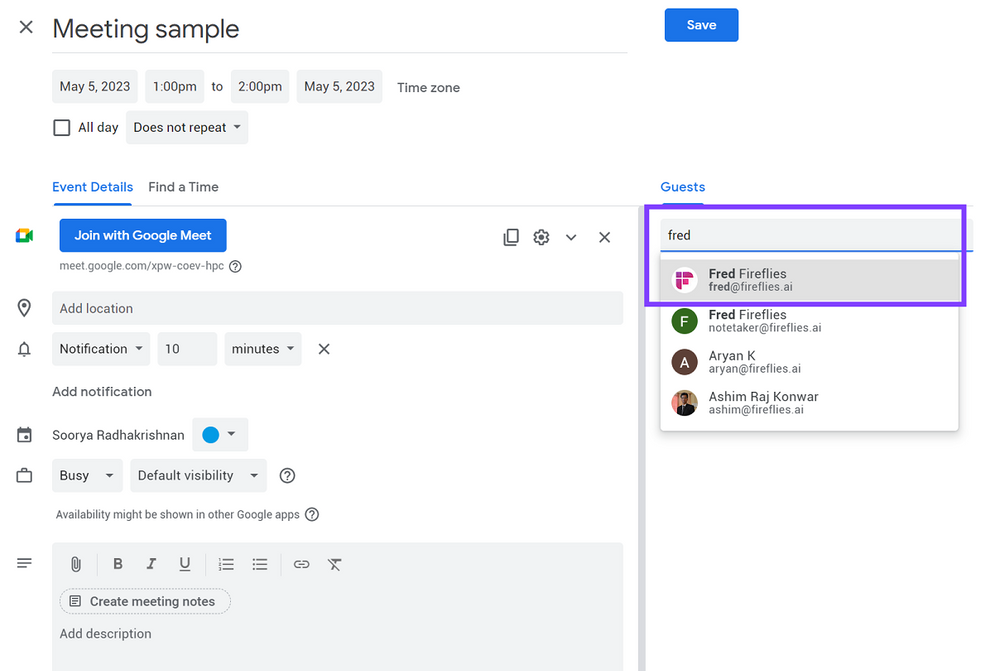The image depicts an event scheduling interface with various elements. At the top, the header reads "Meet and Sample," accompanied by a blue "Save" button. Below this, there's a horizontal line separating the header from the main content. 

The main section features four boxes displaying the event's details:
1. Date: May 5th, 2023
2. Time: 1 PM to 2 PM
3. Time Zone 
4. Unchecked checkbox labeled "All Day"

Next to these boxes, there's a dropdown menu indicating the event does not repeat.

Underneath, the interface displays an "Event Details" section, highlighted with blue, underlined text, and an adjacent option named "Find a Time."

Below these, there's a blue button labeled "Join with Google Meet," followed by a URL: meet.google.com/apw-coev-hpe.

Further down, there's an "Add Location" box and a "Notification" box. To the right of the "Notification" box, it shows the number "10" next to a dropdown menu set to "minutes." Below these elements, there's an option to "Add Notification," and beneath that is the user's name, which is difficult to pronounce.